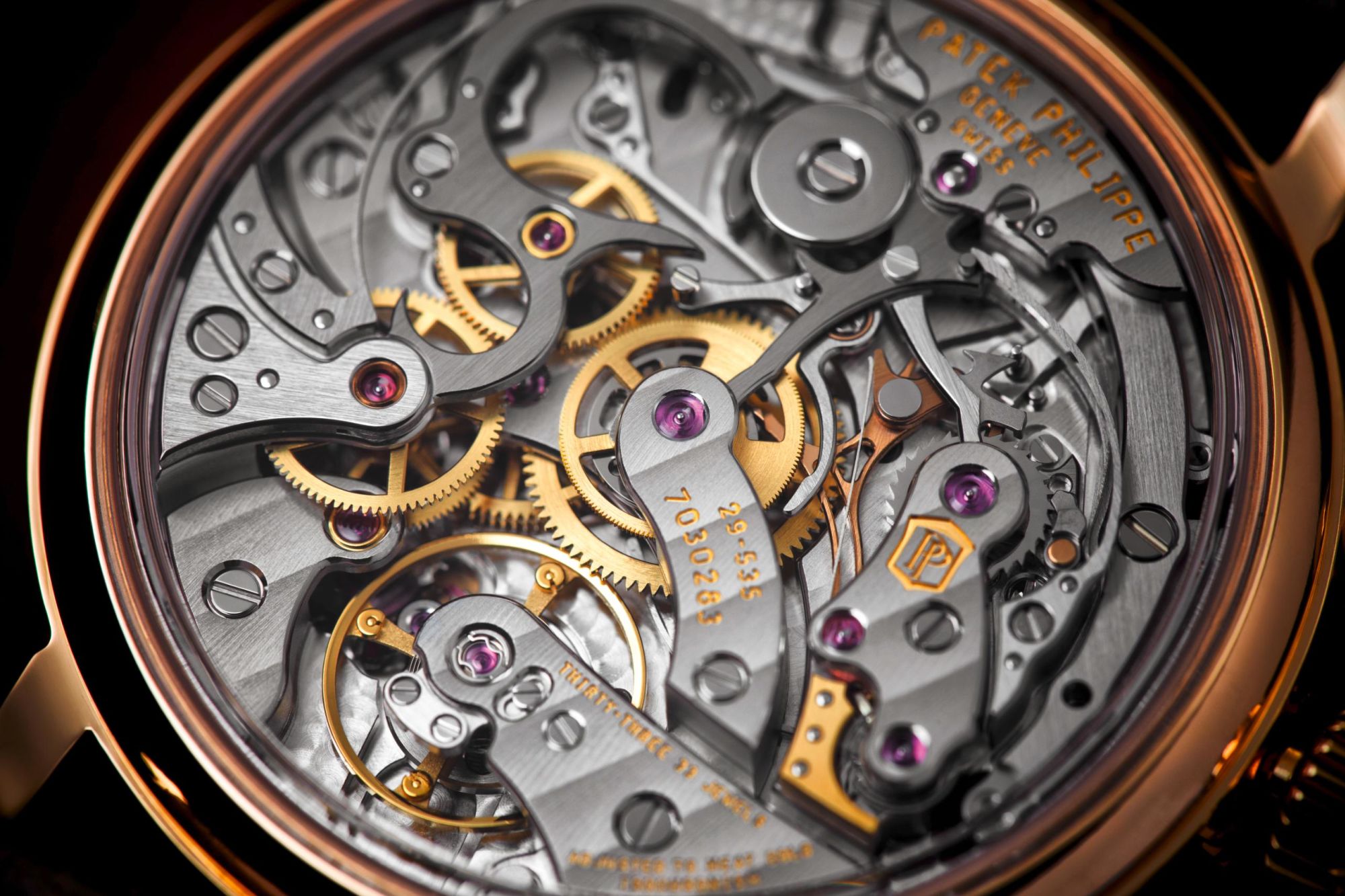This image showcases the intricate inner workings of an expensive, high-end watch. The outer casing forms a copper-hued circle that houses an array of meticulously arranged components. Prominent among these are gold notched gears and shiny silver gears, complemented by parts that appear to be made of dark gray titanium. Various screws are also visible, securing the intricate assembly. Scattered throughout are small, purple dots, whose purpose isn't immediately clear.

In the upper right corner, engraved in reddish-brown font, is the name "Patek Philippe," alongside smaller, less legible text beneath it. The serial number "7030283" is prominently displayed in the middle of the image, emphasizing the watch's unique identity. The craftsmanship suggests exceptional precision and quality, symbolizing the hallmark of luxury timepieces.